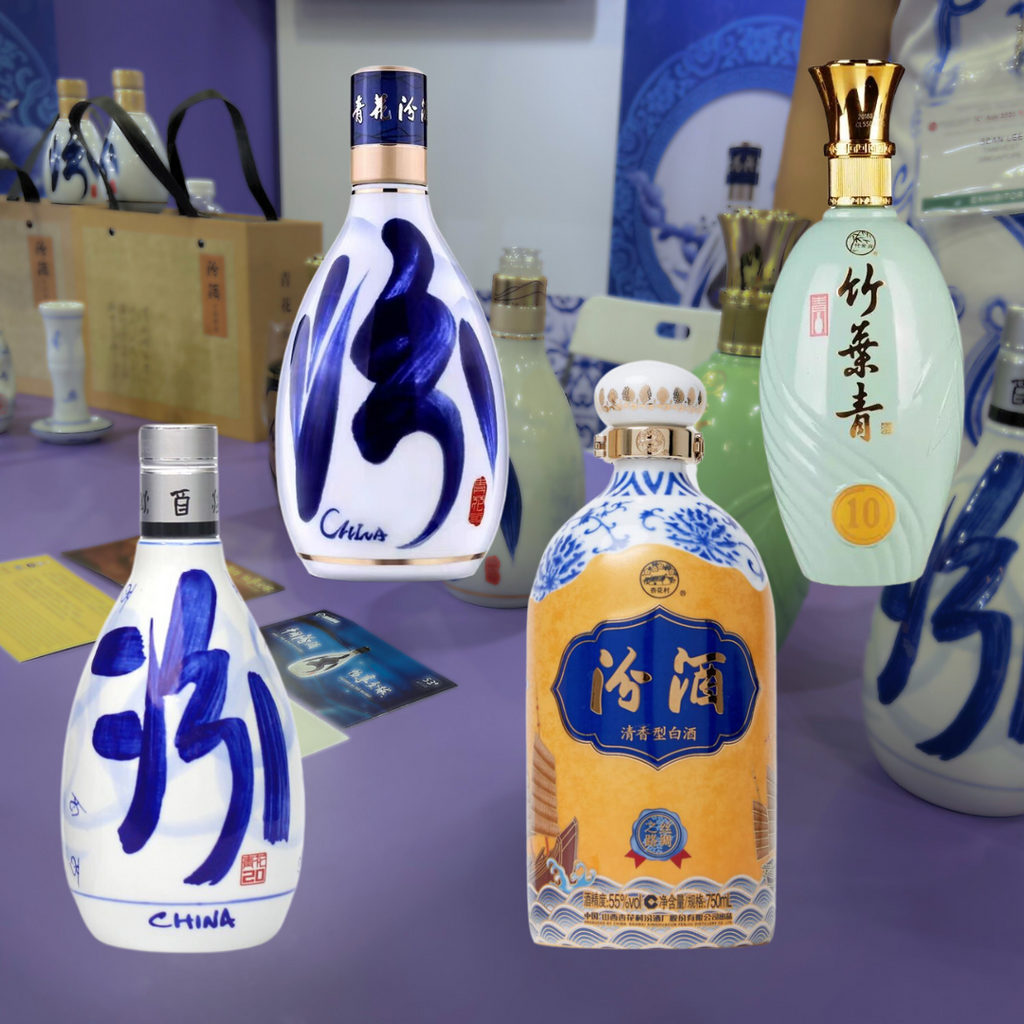The image features an array of bottles containing various types of liquids, prominently displayed in both the foreground and the background. In the forefront, two white bottles with blue labeling and gold neck coverings stand out. One of these bottles has a silver cap, while the other has a blue and gold cap, and both feature Chinese characters and an additional small red stamp.

Adjacent to these, there is a blue and white bottle adorned with a golden label displaying a blue shield and gold writing, as well as a blue ribbon with further gold writing, also in an unfamiliar language. This bottle is topped with a white and gold cap and has red ribbons extending from a medallion-like decoration. Another bottle in the foreground is mint green, featuring black characters in the unknown language and a circular gold sticker marked with the number "10."

In the background, sitting atop a wooden box with a yellow and beige tone and an orange tag displaying more unfamiliar characters, are one or two additional bottles. These background bottles are white with blue labeling and have gold plastic housing over the neck and cap. Further back, there are several more bottles, predominantly green with gold, white, and blue detailing, completing this visually diverse collection.